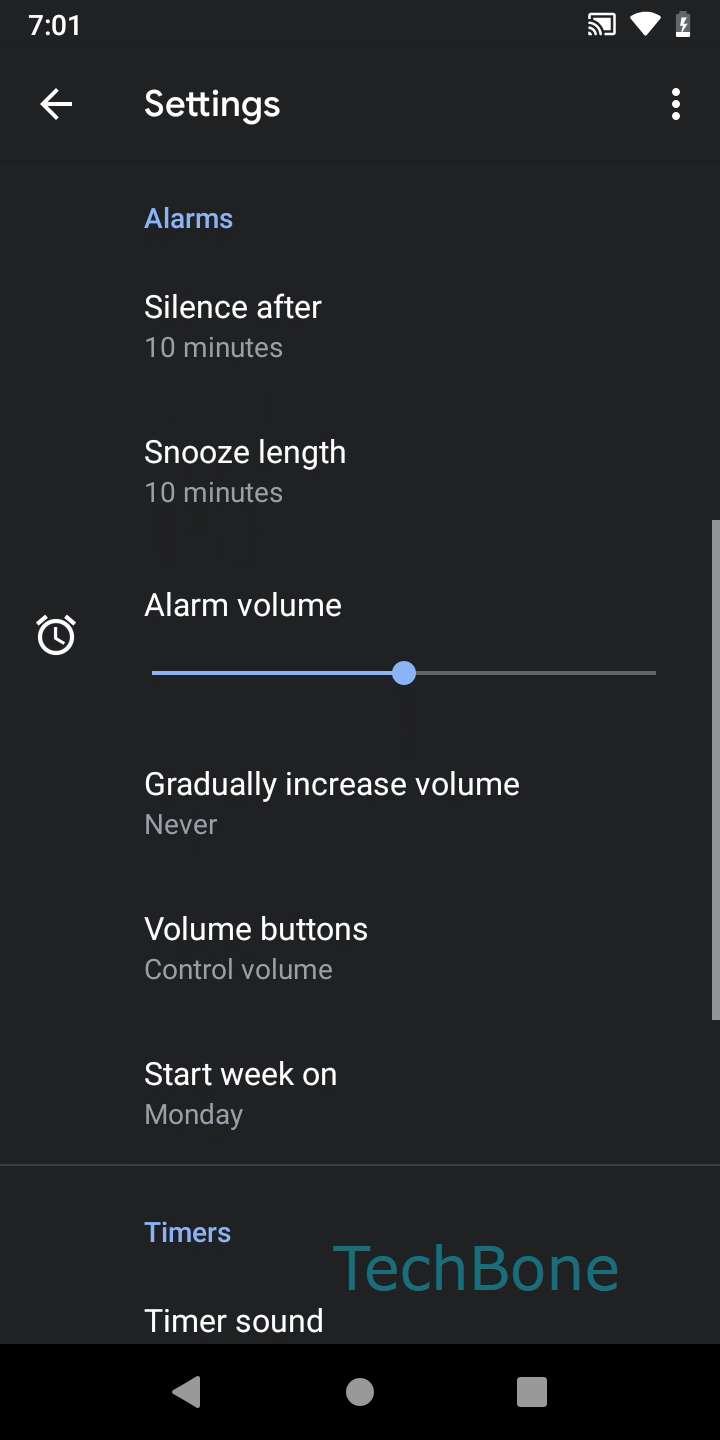This detailed screenshot showcases different elements of a smartphone interface, providing a deep dive into each section's features and appearance.

At the top of the image, there is a thin black border containing various status indicators. On the left, the number "701" is displayed in white text. To its right, there is a screencast icon, represented by a small square with squiggly lines inside. Following this, a Wi-Fi signal icon and a battery icon indicating a low charge are also shown.

Below this border lies a predominantly black background with white text predominantly present throughout the image. In the upper left corner, a white back arrow is visible next to the word "Settings" written in white. Near the upper right corner, a vertical ellipsis (three white dots) is displayed, indicating more options.

Cascading down the screen, a blue text label "Alarms" stands out. Further down, various white text entries detail different options: "Silence after 10 minutes," "Snooze length 10 minutes," and an icon of a small alarm clock labeled "Alarm volume." Adjacent to this, there's a blue slider bar with a blue circle, positioned roughly at the midpoint indicating the current volume setting.

Continuing downward, more setting options include "Gradually increase volume: Never," "Volume buttons control volume," and "Start week on Monday." Below these options, another blue text labeled "Timers" can be found. Subsequently, the white text "Timer sound" is displayed.

Near the bottom, there is a subtle watermark with the text "Tech Bone" in teal blue with a capitalized "T" and "B."

Finally, a black row of icons sits at the bottom of the screenshot, containing a back arrow (triangle), a home icon (circle), and a recent apps icon (square), all depicted in a grayish-white color. The image's quality is high, making all details easily discernible. There are no additional noteworthy elements in this image.